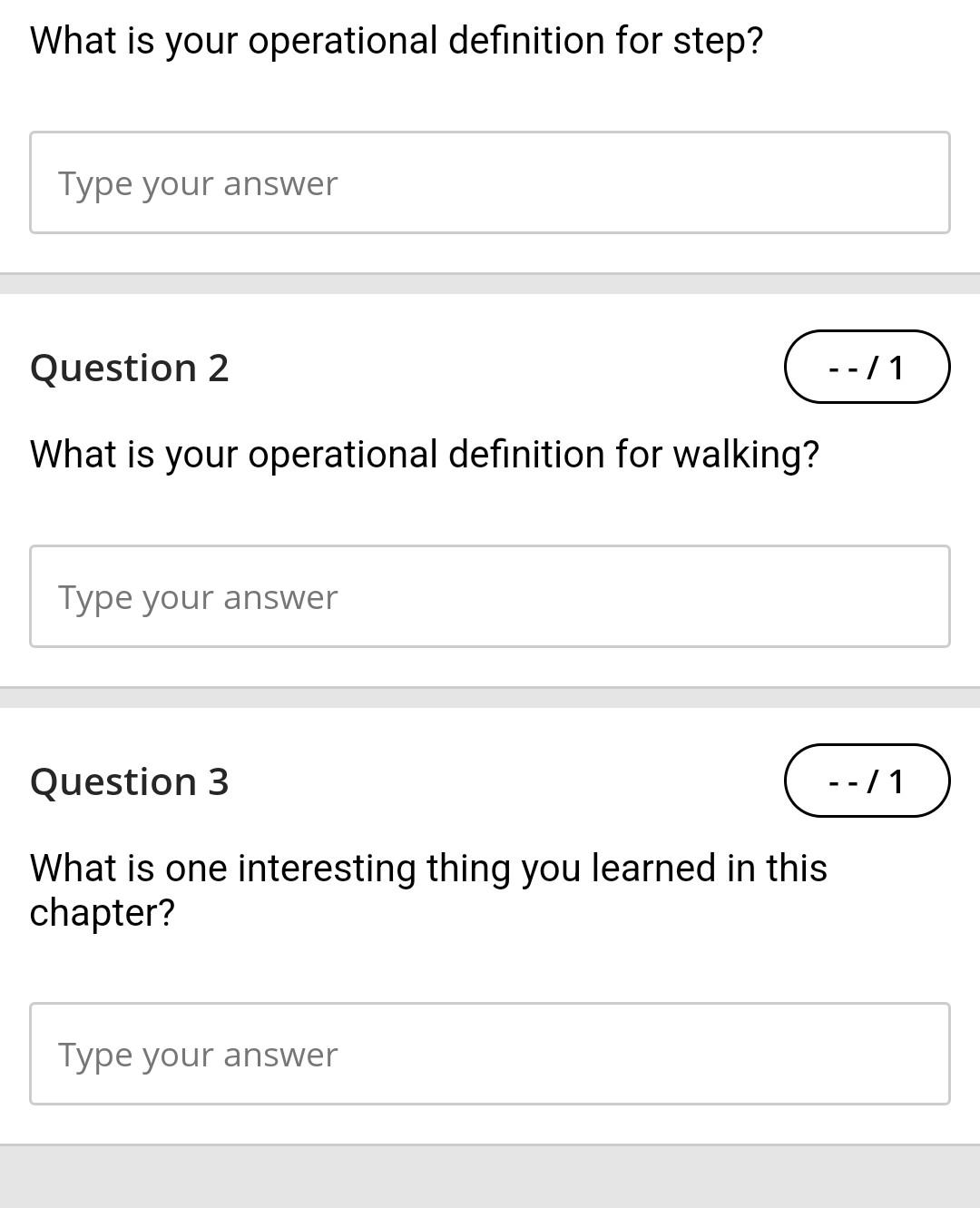The image presents a structured form designed for data organization or as part of a test, featuring clearly defined sections and prompts for user input. At the top of the form, in prominent black letters, it poses the question: "What is your operational definition for 'step'?" Directly below, a light gray-bordered box with a white background invites the user to input their answer, with the text prompt "Type your answer" in light black letters indicating where to type.

A gray line separates this first section from the subsequent one, marked as "Question 2: What is your operational definition for 'walking'?" Above this question, there is an oval icon containing two dashes, a backslash, and the number '1'. Similarly, a gray-bordered box with a white background follows, with the prompt "Type your answer" in light black letters signaling the input area.

Another gray line divides this from the third section labeled "Question 3: What is one interesting thing you learned in this chapter?" This section also features a gray-bordered text box with a white background, accompanied by the prompt "Type your answer" in black letters. Completing the form, a solid gray box lies beneath the last text input area.